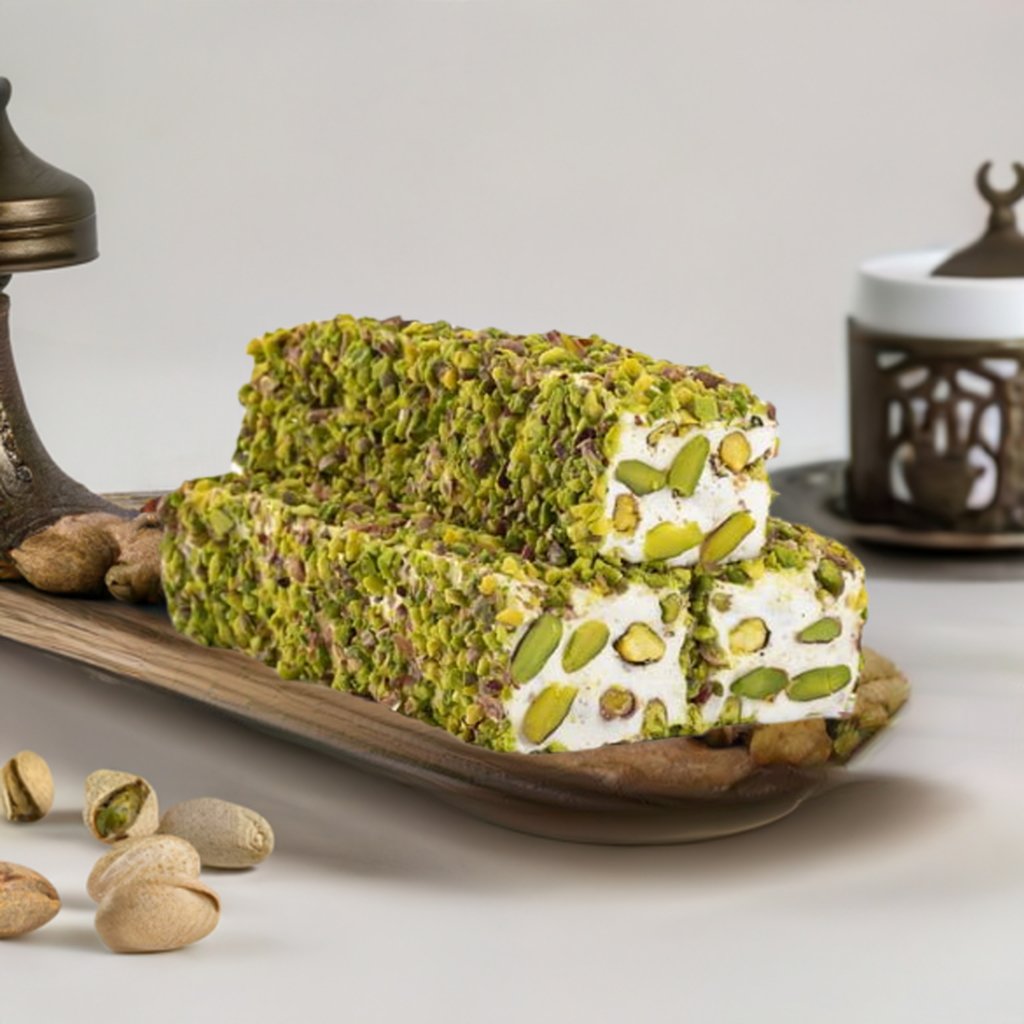The photograph captures three log-shaped pistachio pastries, meticulously stacked with two at the bottom and one on top, displayed on a rustic wooden tray. The pastries are generously coated with finely chopped pistachios, creating a vibrant green and brown exterior, while a marshmallow-like white filling is visible within. For added visual appeal, whole, unshelled pistachios are artfully scattered in the foreground and behind the pastries. In the blurred background, a brass lamp and a white vessel adorned with bronze designs add a touch of elegance to the scene, complementing the earthy tones of the wooden display.